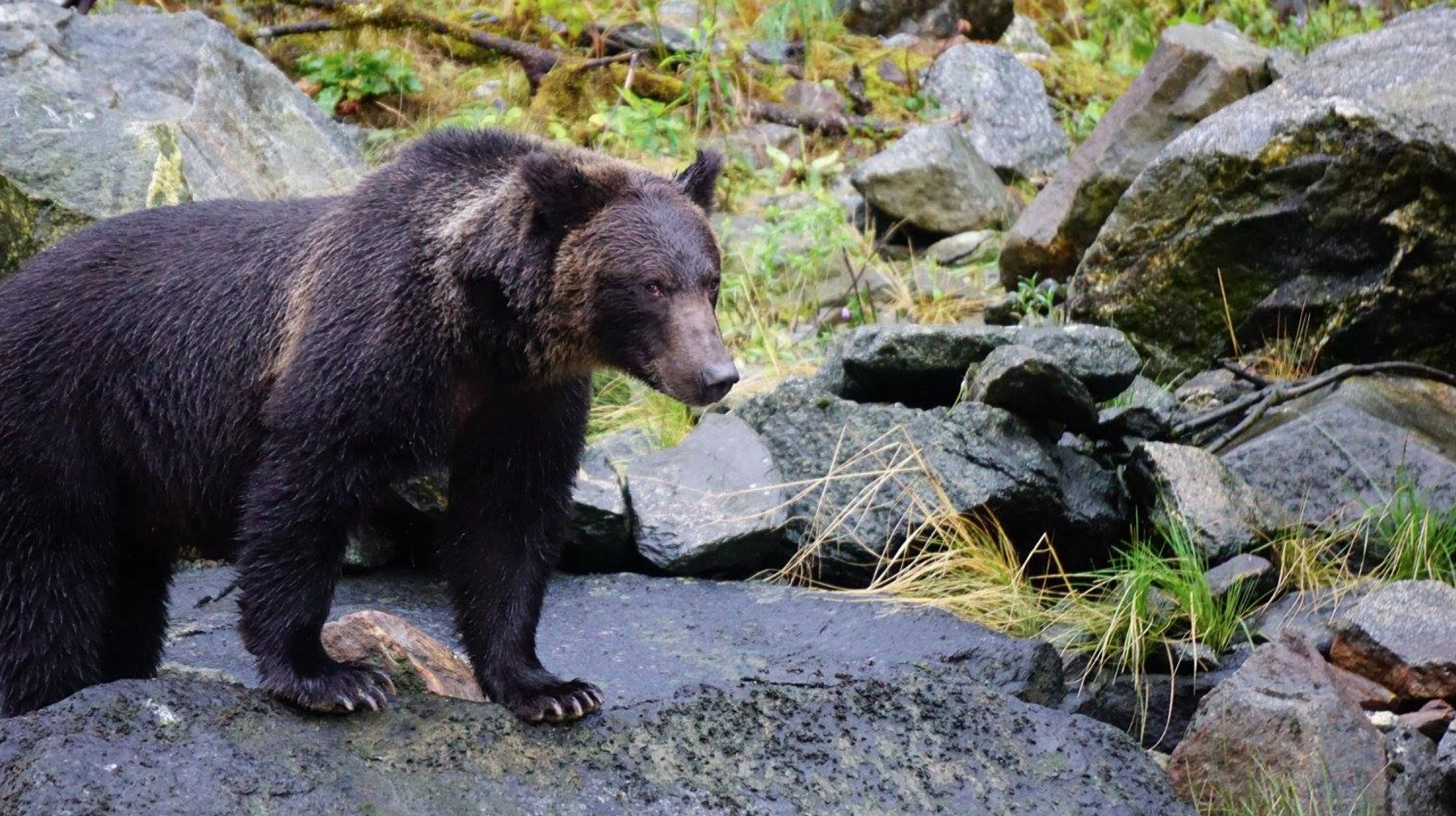The image is a color photograph in landscape orientation, capturing a striking scene of a grizzly bear standing on a rocky hillside covered in large dark gray and black boulders. The bear, positioned on the left side of the image, faces the viewer with its body turned to the right, its front paws slightly spread and gripping a rock. The bear's fur is a deep brownish black color with golden highlights, especially noticeable around its face, which features a long beige muzzle, small rounded ears, and expressive small brown eyes. Its broad shoulders are prominent, and its large beige claws are clearly visible, curled around the front portion of its paws. The backdrop includes greenery, with patches of grass sprouting among the rocks and tree branches scattered across the ground. The setting suggests an outdoor hillside scene, possibly near a cave entrance formed by the piled rocks to the right.